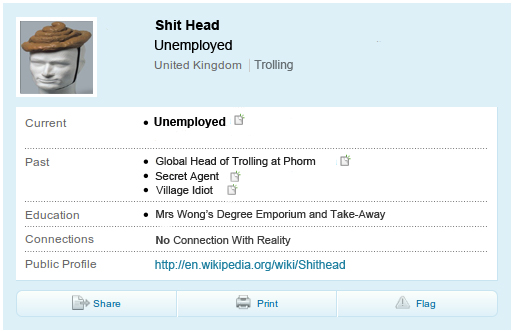The image depicts a satirical, mock online profile card with a light blue background. At the top, the card prominently features a mannequin head wearing a hat resembling a pile of poop secured with a black strap, labeled "SHIT HEAD" in bold letters. The profile details list the individual as "Unemployed," located in the "United Kingdom," and involved in "Trolling." The "Current" status shows them as unemployed, whereas the "Past" roles include "Global Head of Trolling at Forum," "Secret Agent," and "Village Idiot." The education section humorously credits "Mrs. Wong's Degree," "Emporium," and "Takeaway." Under "Connections," it states "No Connection with Reality." Additionally, the "Public Profile" points to a fictitious URL: "wikipedia.org/wiki/SHIT_head." At the bottom of the card, options to "Share," "Print," or "Flag" the profile are provided. The card's absurdity and humorous content clearly indicate it is a joke.